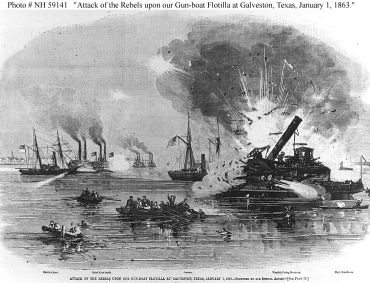This image, seemingly a black and white photograph or an illustration of one, captures a dramatic naval battle scene titled "Photo number NH59141, Attack of the Rebels Upon Our Gunboat Flotilla at Galveston, Texas, January 1, 1863." It appears quite faded, akin to an old postcard. The right side of the image is dominated by a massive explosion on a large boat, with debris scattered across the water. Surrounding the explosion are men in small rowboats, desperately trying to escape, and others who are swimming in the water. The background reveals larger boats, indicative of a gunboat flotilla, with smoke billowing from their engine stacks. Notably, there is also a sailboat present with its sails down. Additional text is visible along the bottom of the image, but it is too small to read.